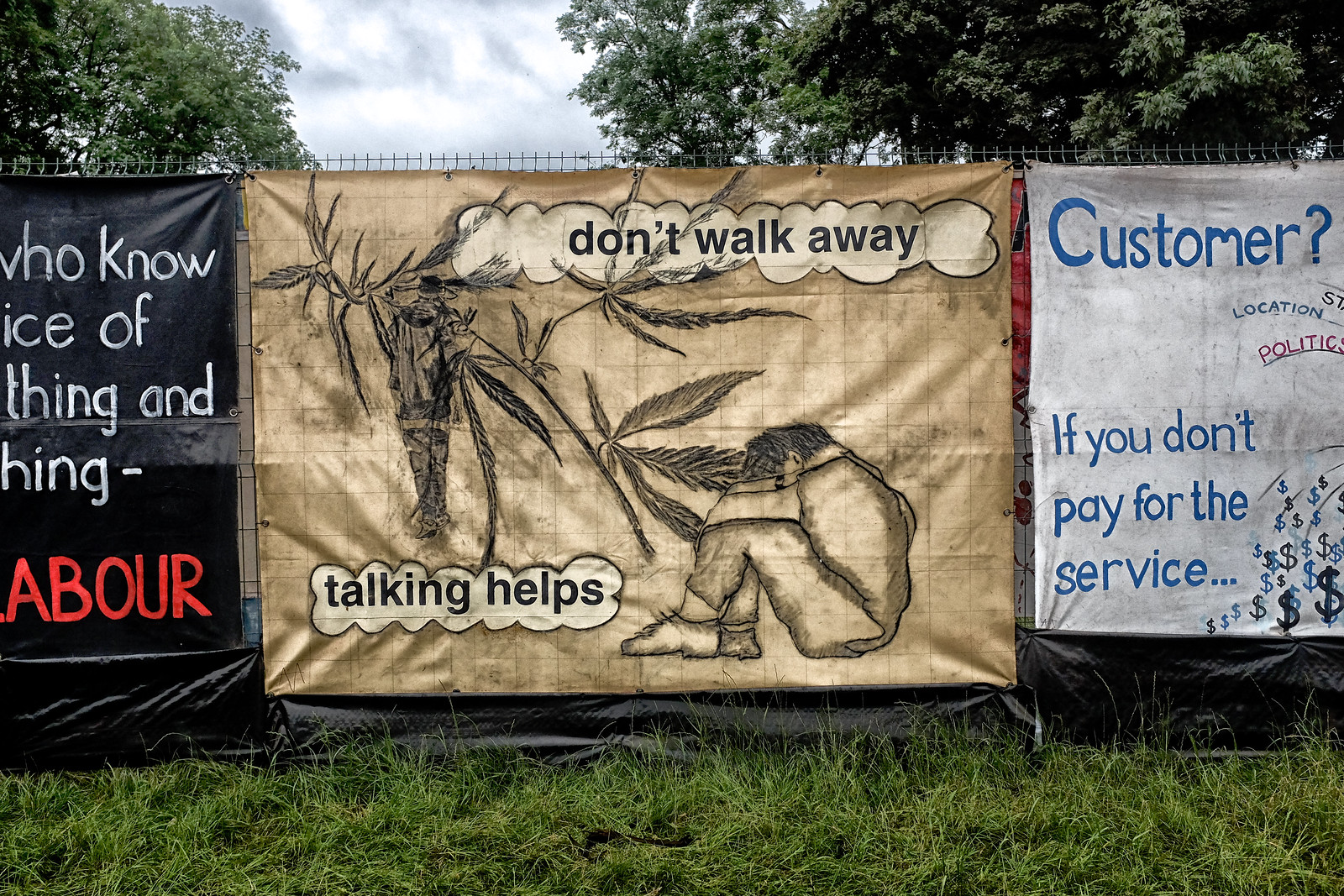The image depicts an outdoor scene with a tall, metal fence featuring many vertical poles and a horizontal bar at the top. The fence stands on a patch of overgrown grass. Three banners hang on the fence. The banner in the middle is brown and features the message, "Don't Walk Away," with "Talking Helps" written beneath it. This central banner includes an artwork of a person, appearing distressed, sitting with their knees bent and their face buried in their hands, surrounded by brown leaves. The banner on the right is partially visible and is black. Beyond the fence, lush green trees and a blue sky with white clouds form the backdrop. The overall scene suggests themes of mental health and social activism.